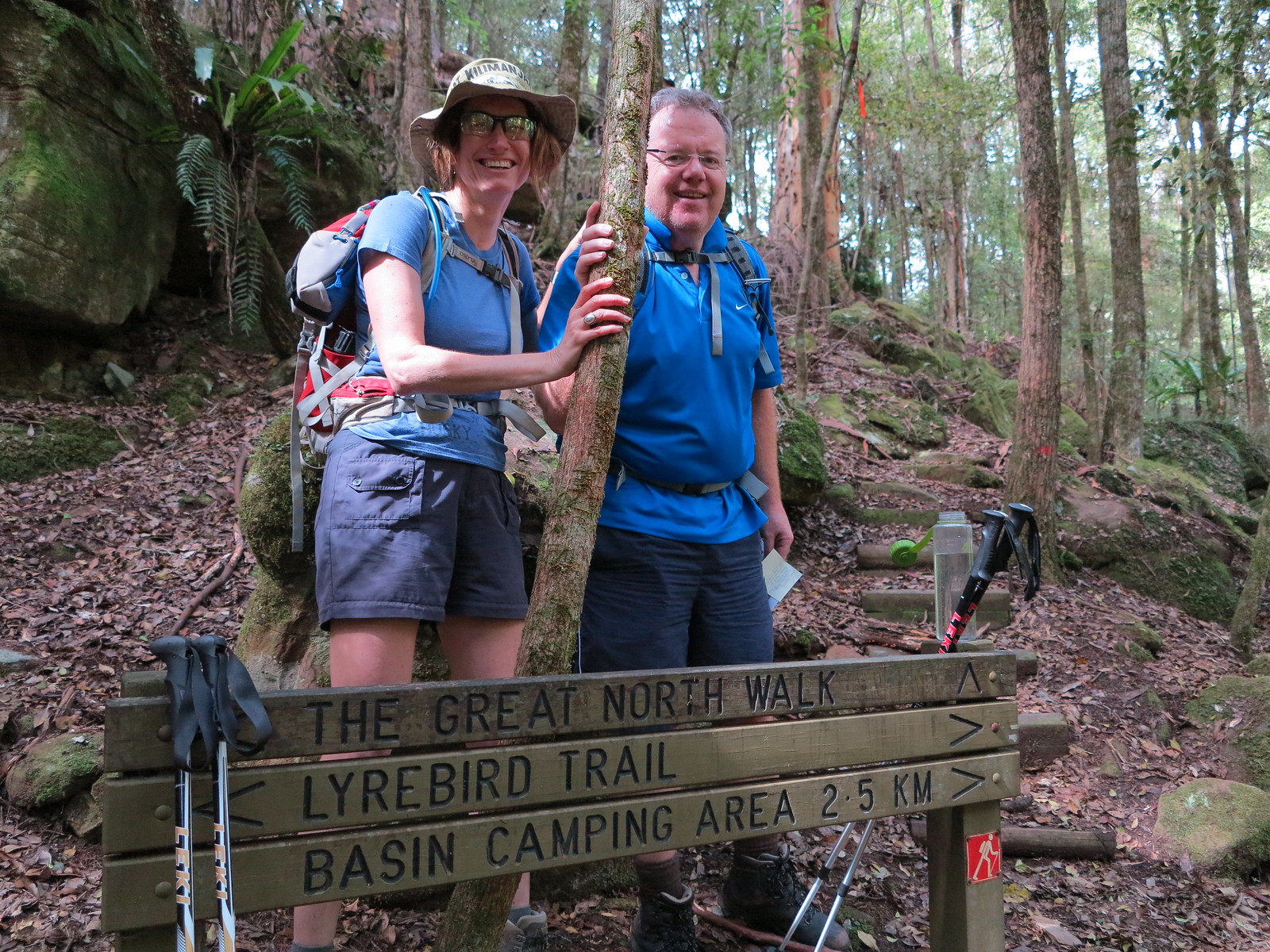This photo captures a scenic moment in a woodland setting featuring two individuals, a woman and a man, posing in the center of the frame. Both appear to be prepared for an outdoor adventure, dressed in camping gear rather than for a casual walk. The woman on the left, identified as Finn, is equipped with goggles, a brown khaki hat, a blue t-shirt, black shorts, and a red backpack. Her backpack features straps around her waist and chest, and a blue hydration pipe. She stands smiling, gripping a tree. To her right, the man is also dressed in a blue shirt, shorts, and glasses, with similar backpack straps around his body. He too smiles at the camera while holding onto the tree.

At their feet is a wooden sign comprising three horizontal bars. The top bar reads "Great North Walk" alongside a black carved owl, accompanied by an upwards-pointing arrow. The second bar indicates the "Lyrebird Trail" with arrows pointing left and right. The bottom bar informs that the "Basin Camping Area" is 2.5 km ahead, with an arrow directing to the right. In front of this sign rest two walking sticks, while two more lean on the posts behind it. A water bottle with its lid unscrewed lies just to the left of the walking sticks.

The surrounding environment looks partly tropical, featuring dense vegetation, trees, and a large rock on the left of a set of steps leading upward. The area is bathed in daylight, with clear skies overhead, giving the impression of an inviting, serene hiking trail through lush trees.